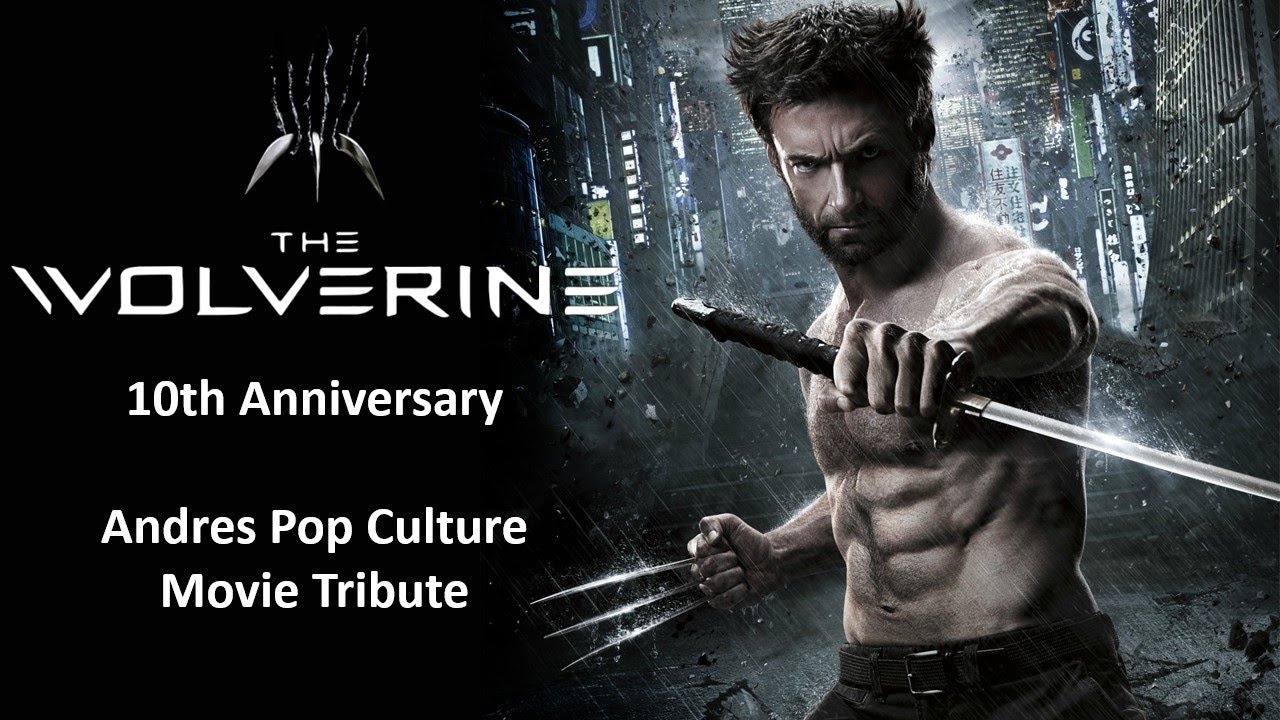This poster commemorates the 10th anniversary of the movie "The Wolverine." On the right side, a dynamic illustration features Hugh Jackman as Wolverine, shirtless with black pants and a belt visible from the waist up. He faces the camera intensely, with a long sword in his left hand and the iconic Wolverine claws extended from his right knuckles. His rugged appearance is completed by his short brown hair and beard. The backdrop is a dystopian cityscape with densely packed buildings and glowing neon signage, evoking a Japanese urban environment.

On the left side of the image, a stark black background prominently displays the text in large white letters: "The Wolverine, 10th Anniversary, Andres Pop Culture Movie Tribute." Above this text, a Wolverine logo adds to the tribute’s celebratory theme.